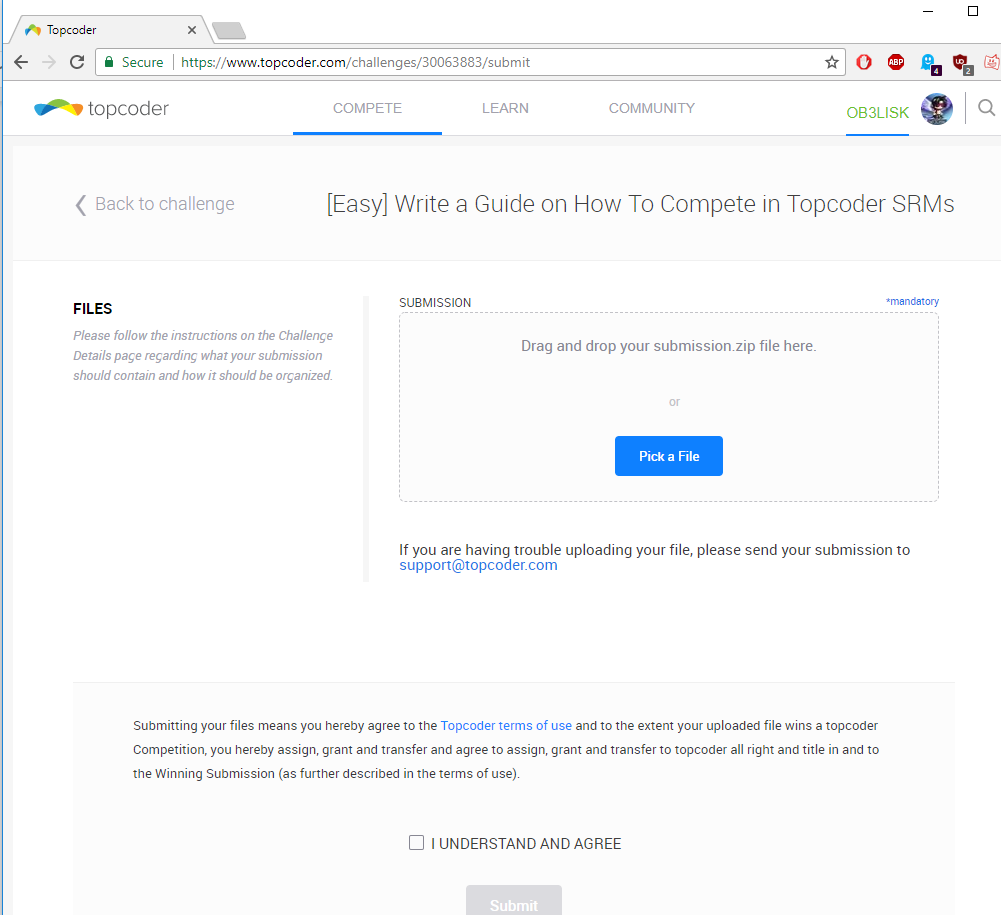The image depicts a user navigating the TopCoder website. In the search bar at the top of the browser, the URL "www.topcoder.com" has been entered. The page displayed is the homepage of TopCoder, which features the TopCoder logo—a small, multi-colored squiggly line in shades of yellow, orange, green, and blue. 

Beneath the logo, there are three key sections: "Compete," "Learn," and "Community," with "Compete" prominently underlined. A highlighted section on the page indicates an instructional guide titled "Write a Guide on How to Compete in TopCoder SRMs (Single Round Matches)." 

To the left, a navigation link labeled "Back to Challenge" is visible. Below this, there is a section titled "Files," with a directive to follow the instructions on the Challenge Details page regarding submission content and organization.

At the center of the page, there is a submission interface with a prompt that reads "Drag and drop your submission .zip file here" and an alternative "Pick a file" button, highlighted in blue. Underneath this, there is a legal disclaimer stating that "Submitting your files means you hereby agree to TopCoder's terms of use. To the extent your uploaded file wins a TopCoder competition."

Finally, a checkbox with the statement "I understand and agree" needs to be checked before the gray "Submit" button can be activated.